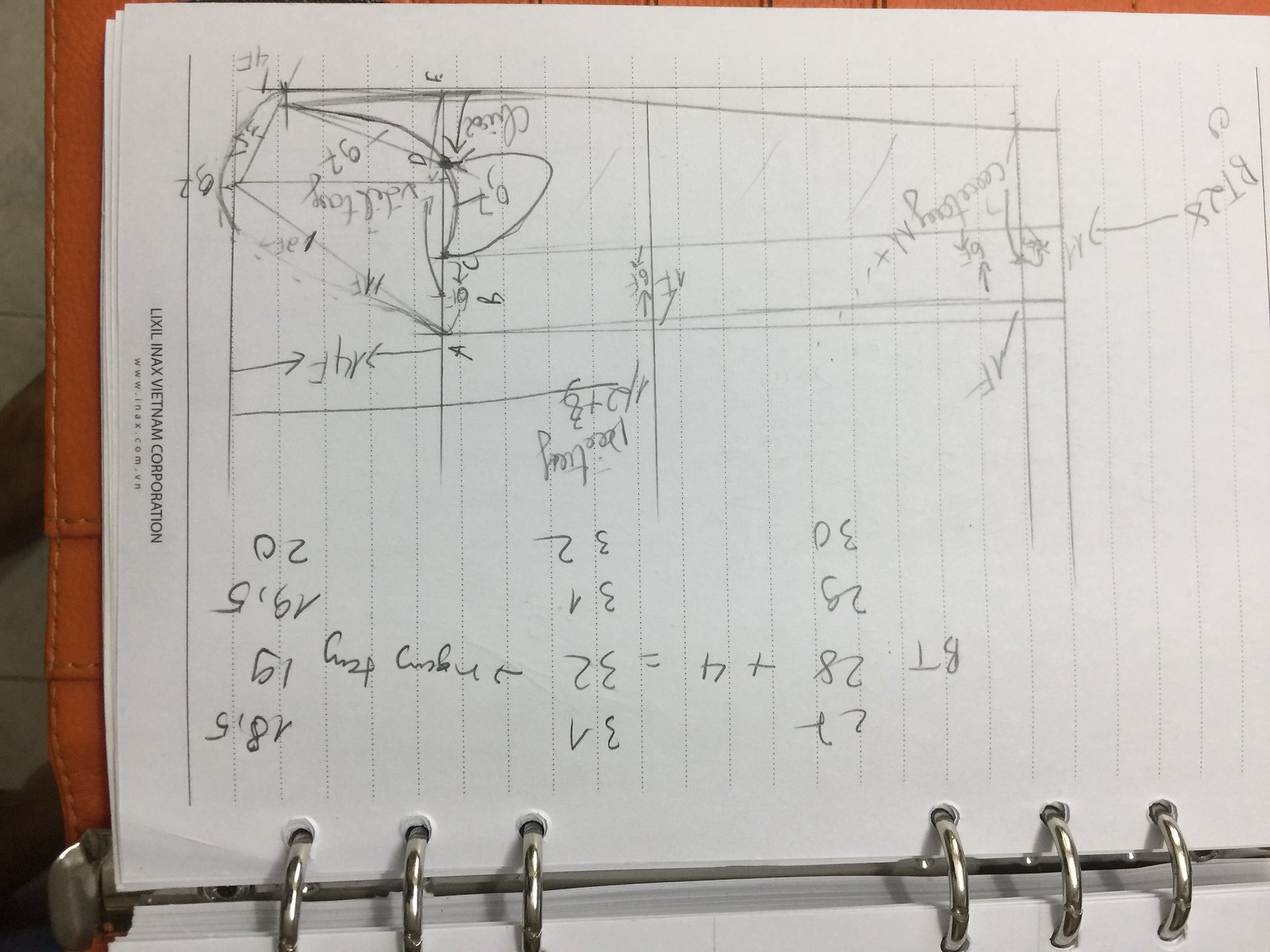This is an image of a refillable journal with a brown leather-like cover. The journal is oriented such that viewers see it from the side, highlighting its binder rings, which allow for the easy addition and removal of pages. The opened page prominently displays text at the bottom, including the words "Vietnam Corporation" followed by names that are difficult to pronounce. The page itself is lined, with various structured elements at the top, such as lines, squares, and charts containing a mix of numbers and symbols, some representing measurements. Additionally, the page features various numeric values and calculations, including a detailed entry "BT, 28 + 4 = 32."